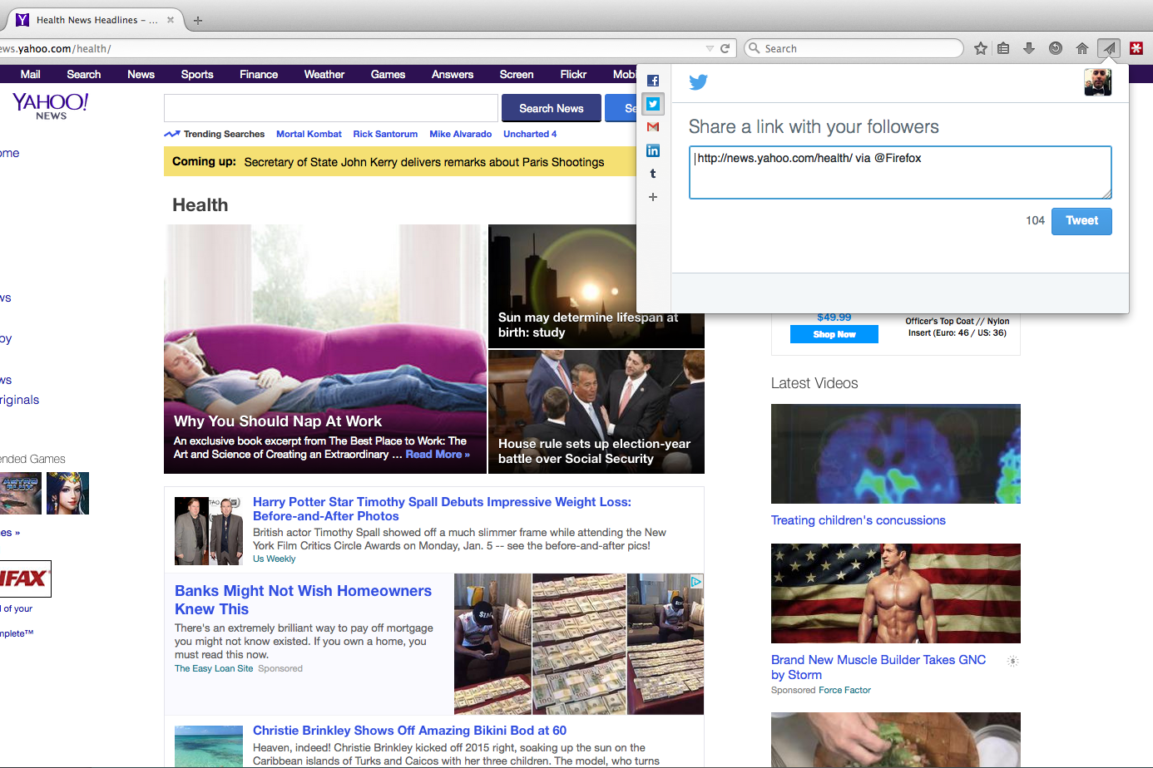The image depicts a Yahoo website interface displayed on a computer screen. At the top, the page features a familiar Yahoo header with a noticeable purple square and some indistinct letters. Directly below is the address bar, displaying "yahoo.com" followed by an unreadable section. Beneath the address bar, a prominent purple navigation bar contains text and a search functionality labeled "Yahoo News." An outlined gray rectangle acts as the search input field, designed for users to enter their queries, accompanied by a "search news" button.

Further down, the page contains a mix of news highlights and features. A yellow rectangle stands out, announcing an upcoming segment titled "Secretary of State John Kerry delivers remarks about Paris shootings." Adjacent to this, an image of a man lounging on a couch accompanies an article titled "Why you should nap at work," with additional, unreadable text below.

The website also shows a partially visible image of a sunlit cityscape and an older photograph of Congressional members in session. Two smaller, indistinct images follow along with a headline about "Harry Potter" star Timothy's impressive weight loss, showcasing before and after photos. Another story title, barely legible, reads "Banks might not wish homeowners knew this," next to images that appear to be related to home repairs. A feature on Christie Brinkley mentions her stunning bikini appearance at 80.

On the sidebar, there is a white section highlighting social media sharing options, with the blue Twitter bird icon at the top. Other social media icons are positioned to the left. The caption "Share link with your followers" appears with an accompanying link and a "tweet" button in a small blue box.

At the bottom, the section labeled "Latest videos" includes a blend of colored rectangles: blue, purple, and green hues, followed by an American flag with a shirtless person standing in front of it. The text caption here discusses "Treating children's concussions," and another video headline states "Brand-new muscle builder takes GNC by storm."